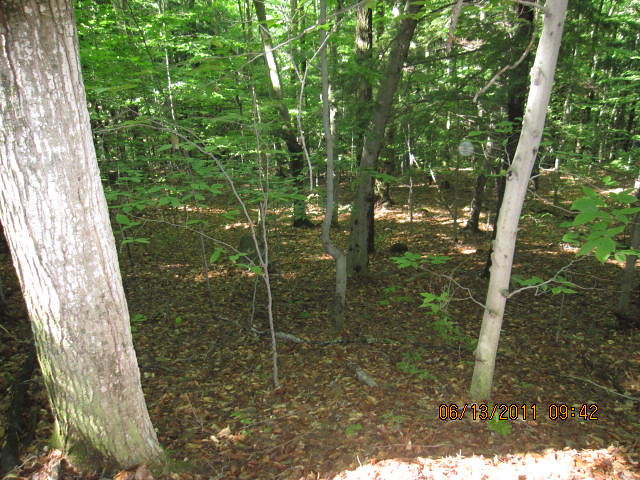The photograph is a rectangular outdoor shot taken in a heavily wooded area during the morning of June 13, 2011, as indicated by the orange time and date stamp "06 13 2011 09:42" in the bottom right corner. The image captures a forest primarily consisting of young, thin, bright green maple trees, with their leaves freshly blooming. The ground is layered with a thick carpet of brown, decaying leaves, interspersed with small plants and possibly patches of poison ivy. A distinctive large tree with a thicker trunk stands prominently to the far left, contrasting with the otherwise uniformly slender trees. Sunlight filters through the canopy, casting bright patches on the leaf-covered ground and highlighting the trees' trunks and branches, further confirming that the photograph was taken in the morning. The forest scenery suggests an environment typical for hiking trails, full of natural growth and subtle underbrush.